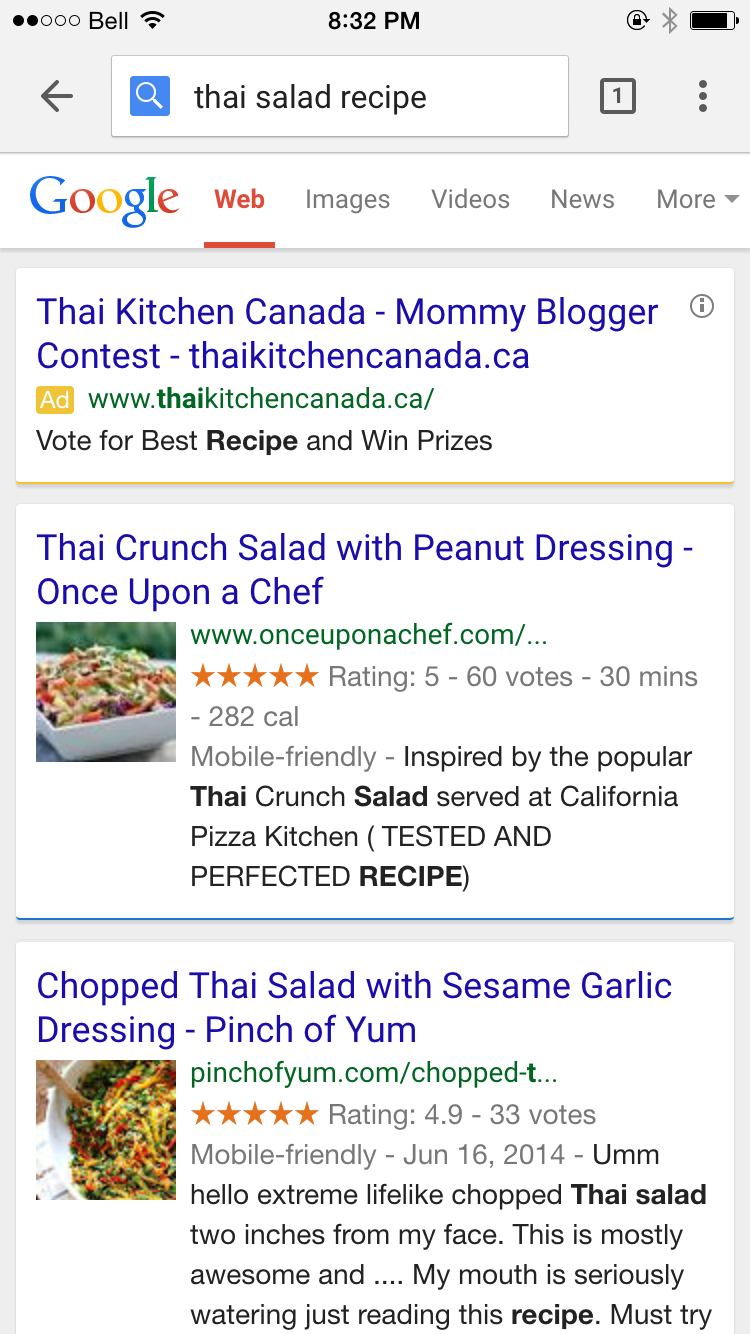This image is a detailed screenshot from a tablet taken at 8:32 p.m., connected to the Bell Network with nearly a full battery. The tablet user is conducting a Google search for a "Thai salad recipe." The Google search interface highlights the "Web" tab in red, while other options such as "Images," "Videos," "News," and "More" are in light blue.

Below the search bar, three web search results are displayed:

1. **Thai Kitchen Canada Mommy Vlogger Contest** (Ad)
   - **Website:** www.ThaiKitchenCanada.ca
   - **Description:** "Vote for best recipes and win prizes."

2. **Thai Crunch Salad with Peanut Dressing - Once Upon a Chef**
   - **Website:** www.onceuponachef.com
   - **Rating:** Five stars with 60 votes
   - **Details:** "30 minutes, 282 calories"
   - **Notes:** A highly-rated, mobile-friendly recipe inspired by the popular Thai Crunch Salad served at California Pizza Kitchen, shown with a white serving tray filled with food.
   
3. **Chopped Thai Salad with Sesame Garlic Dressing - Pinch of Yum**
   - **Website:** www.pinchofyum.com/chopped
   - **Rating:** 4.9 stars with 33 votes
   - **Details:** Mobile-friendly, posted on June 16, 2014
   - **Notes:** Contains a white bowl with the salad and chopsticks, described as extremely lifelike and mouth-watering, prompting a must-try.

Each search result provides key information such as ratings, preparation time, calorie count, and visual thumbnails of the dishes.